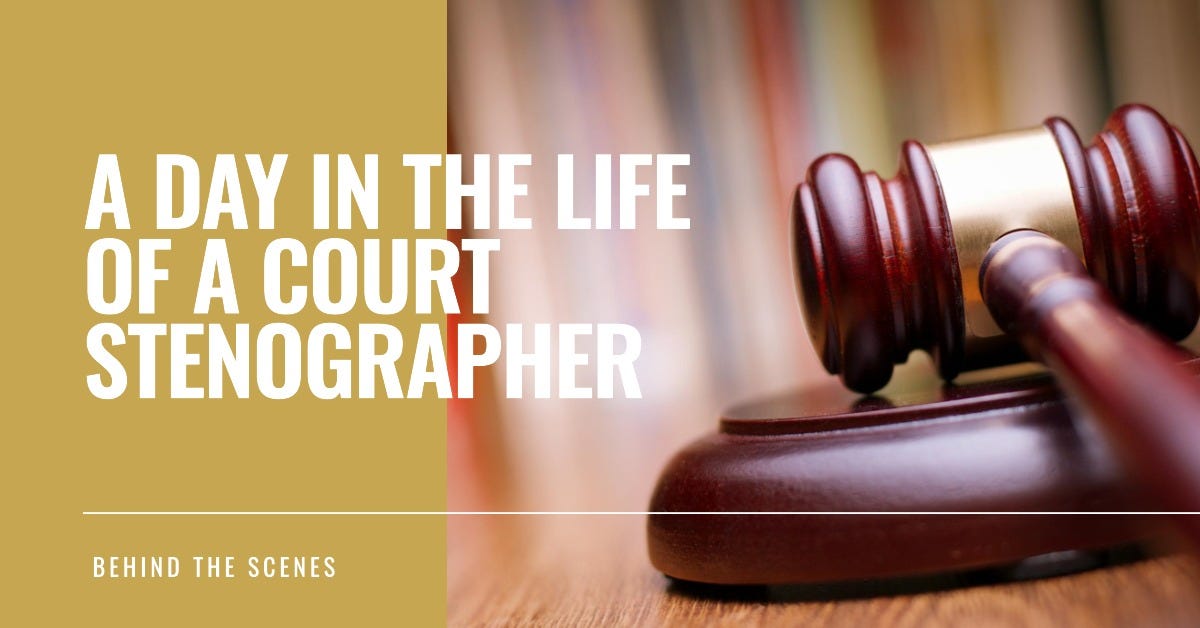The image appears to be an advertisement featuring a judge's gavel, crafted from rich mahogany with a gold band at the handle-hammer junction, resting on its circular strike pad atop a wooden table. The background is blurred with reddish and yellow hues, adding depth and focus to the gavel. On the left side of the image, there is a solid beige rectangle with large, white block letters reading "A Day in the Life of a Court Stenographer." Below, in smaller white text, it says "Behind the Scenes," separated by a thin horizontal white line extending almost across the entire image. The design is eye-catching yet simple, effectively drawing attention to the subject matter—an insightful ad intending to showcase the behind-the-scenes role of a court stenographer.